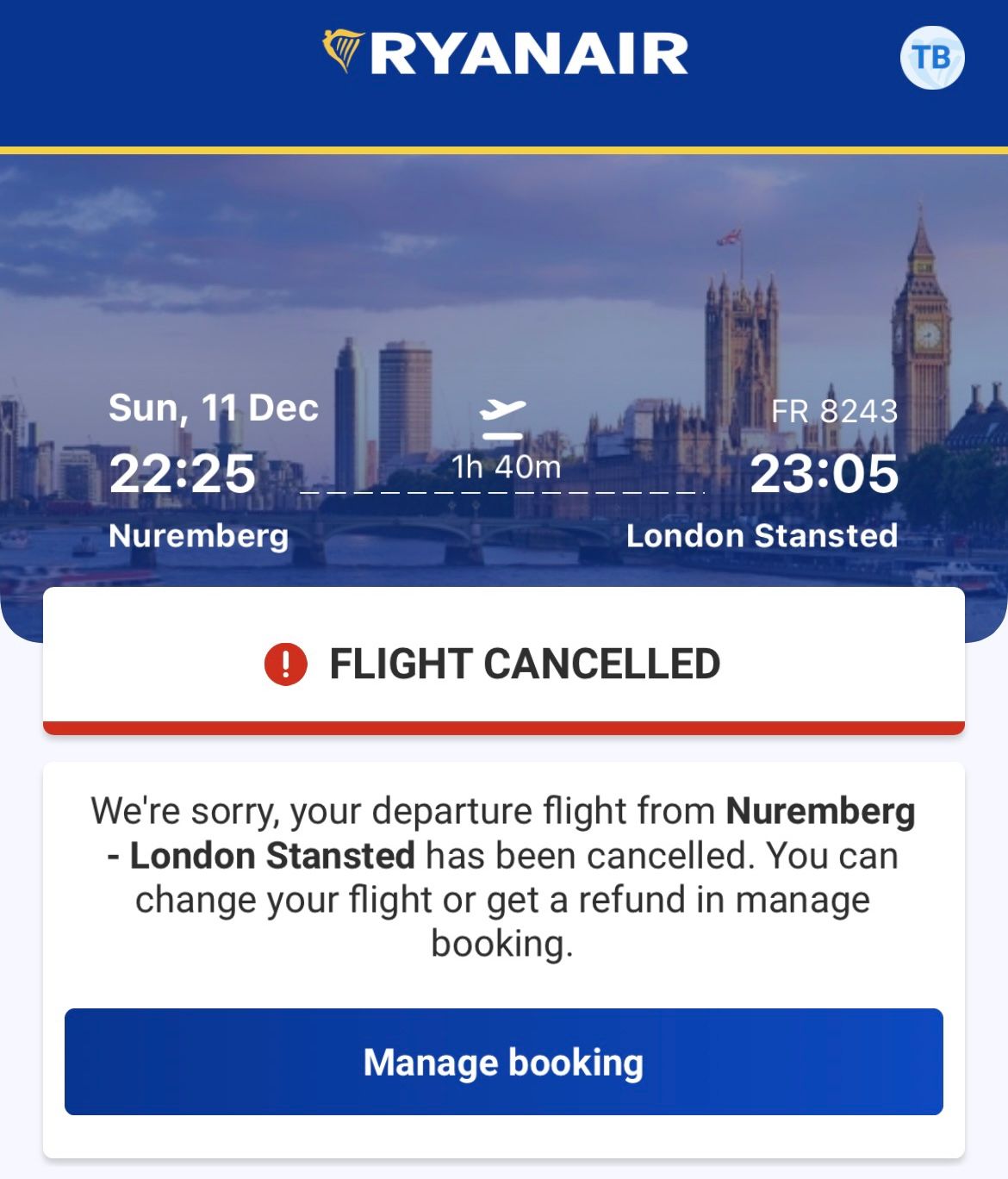This is an image of the Ryan Air website, showcasing information about a flight. The interface features a blue background and prominently displays a photo of a cityscape, likely London, with several tall buildings and clouds visible in the background. At the top of the image, 'Ryan Air' is written in bold white letters, accompanied by a bird icon with striped wings on the left side of the 'R'. To the right of this logo, the letters 'TB' are enclosed in a white circle.

Within the central image, the flight information is detailed. The date 'Sunday, the 11th of December' and the time '22:25' are displayed. At the bottom, 'Nuremberg' is written in white text. The middle part of the image features an illustration of an airplane taking off, aligned with a line indicating a duration of '1 hour and 40 minutes', accompanied by dotted lines below it. Additional times 'Friday, 8:24', '2305', and the destination 'London Stansted' are noted.

At the bottom, there is a white square with the text 'Flight Cancelled' in black. Below, a white background section contains a red circle with a white exclamation point on the left-hand side. The message, in bold black text, reads: "We're sorry, your departure flight from Nuremberg to London Stansted has been canceled. You can change your flight or get a refund and manage booking." A blue rectangular button labeled 'Manage Booking' is situated at the bottom, providing an option to press for further action.